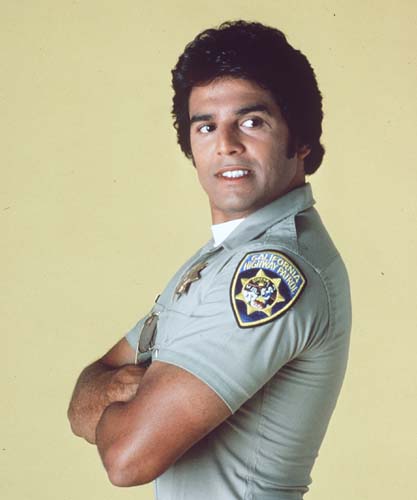This photograph captures actor Eric Estrada in his iconic role as a police officer from the classic TV show "CHiPs." Estrada, a Latino male with dark, slightly wavy hair that curls over his left ear, is clad in a tan California Highway Patrol uniform. This outfit features a gold star-shaped badge on his left chest, and a patch on his left shoulder indicating his department. His bright white teeth are visible in a composed, yet slightly happy, smile, suggesting a serious demeanor infused with a hint of warmth. Estrada stands with his arms folded across his chest, his body oriented towards the left side of the photograph while his gaze is directed to the right. His black sunglasses dangle from his right arm. The background behind him is a muted yellow, highlighting the era and style of the old promotional shot.